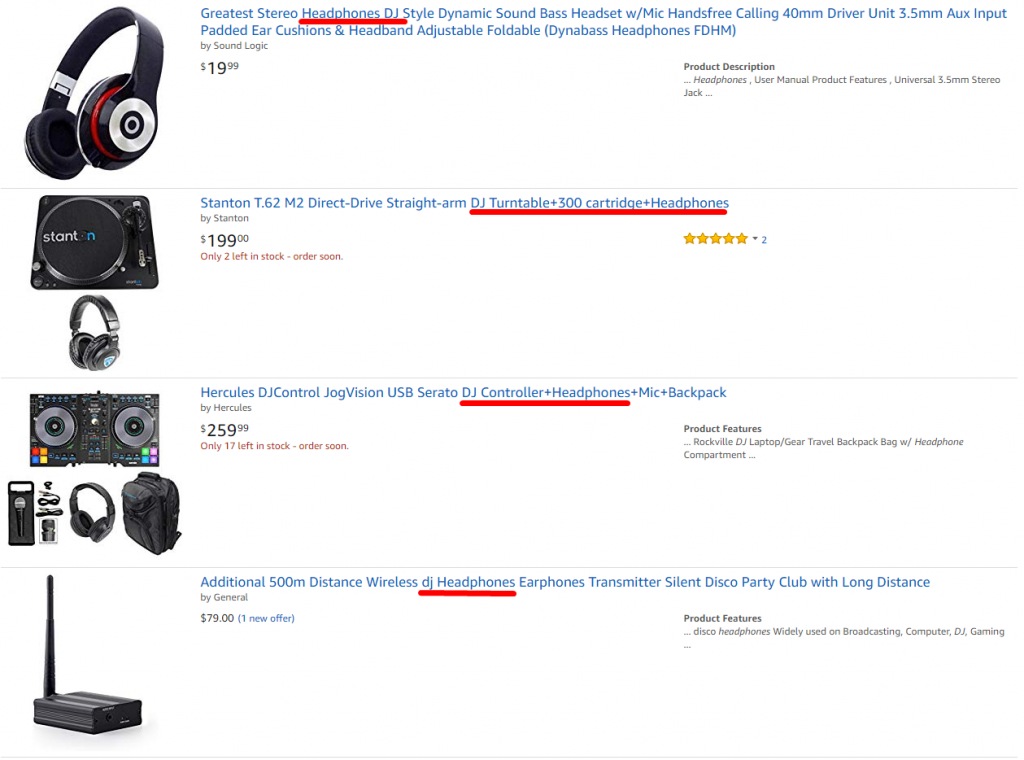This screenshot from Amazon displays a selection of DJ-related products. At the top is a pair of black and red over-the-ear headphones, labeled "Headphones DJ" in red underlined text, priced at $19.99. Below it is a "DJ Turntable plus 300 Cartridge plus Headphones" package, priced at $199. The turntable is designed for DJs, suitable for vinyl scratching and mixing. This product has a rating of five stars from two reviews.

The third product, titled "DJ Controller plus Headphones" in red underlined text, includes a DJ controller, headphones, a microphone, and a backpack. This comprehensive DJ setup is priced at $259.99. 

At the bottom, the final product is labeled in red underlined text as "DJ Headphones." However, it is actually an extender kit for wireless DJ headphones, titled "Additional 500 Meter Distance Wireless DJ Headphones, Earphone Transmitter, Silent Disco Party Club with Long Distance." This product is specifically designed for long-distance, wireless audio transmission.